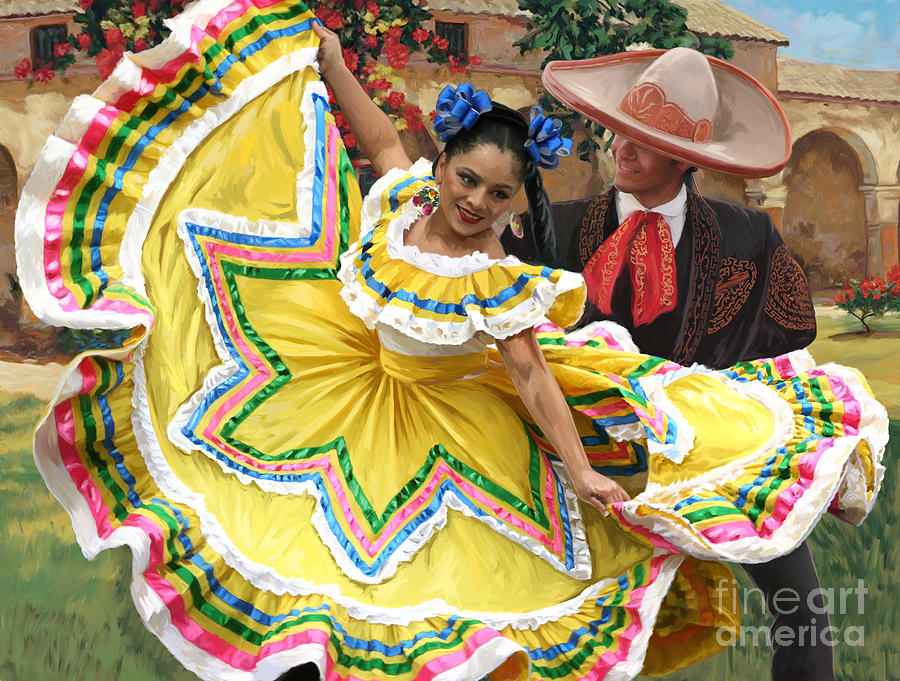The artwork is a colorful, detailed painting of two people dancing in traditional Latin American attire in a grassy area in front of a beige, painted stone house adorned with flowers and vines. The scene includes a bit of blue sky with white clouds in the upper right corner. The woman, positioned on the left, is wearing a vibrant, puffy yellow dress with intricate patterns in white, green, pink, and blue, and she has blue bows in her black braided hair. She holds up the hemline of her dress with both hands, smiling brightly while displaying dark red lipstick and large earrings. The man stands slightly behind her to the right, dressed in a black suit with gold accents, a large brown sombrero with orange trim, and a red and gold ribbon tied at his neckline. The image captures the essence of festive Latin American culture with its vivid colors and dynamic composition, and the lower right corner is marked with "Fine Art America."